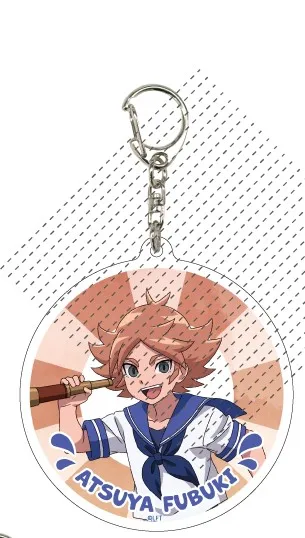The image showcases a keychain featuring a circular fob displaying an anime-style character with medium-length, chestnut wavy hair. The character, identified as Atsuya Fubuki, is dressed in a blue and white sailor outfit, complemented by a handkerchief tied around the neck. He holds a spyglass in his right hand. The background of the key fob resembles a life ring with white and tan patches, and it includes the name "Atsuya Fubuki" inscribed at the bottom in blue text. Additionally, the design is accentuated by black dotted lines that run diagonally across the image, creating a watermark effect that partially obscures the underlying illustration. The overall palette is enhanced by subtle water droplet decorations.